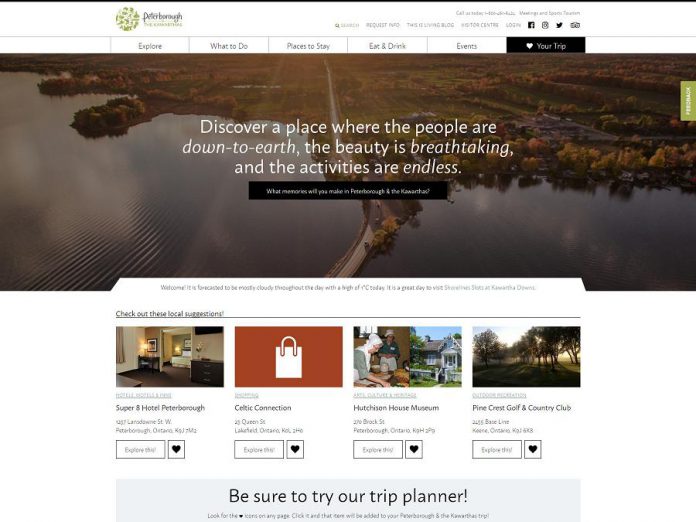The image features a complex and layered design with a mix of graphical and textual elements. Starting from the top:

A thin gray line spans horizontally across the image, blending with darker shades of gray, black, or possibly navy blue, making it hard to discern the exact color. 

On the left side, there's a circular emblem composed of green and white elements that are indistinct upon zooming in. This emblem might depict animals, though clarity is lost when zoomed. Adjacent to the emblem, the text "Peter's Barrel" appears in black, followed by an indistinct green text below it.

To the right, the text "request info" appears in black, followed by an unreadable word that ends with "blog." Continuing to the right, there is centered text reading "login."

Below are various bordered tabs:

1. Explore
2. What to Do
3. Places to Stay
4. Eat and Drink
5. Events

The first five tabs have a white background with black text. A sixth tab, set against a black background, features a white heart icon and the words "your trip."

Dominating the central part of the image is an aerial view that includes a sunrise casting a warm glow over trees and dark-colored water. Superimposed on this scenic backdrop is the text: "Discover a place where the people are down to earth. The beauty is breathtaking, and the activities are endless." Below this, a black rectangle contains partially visible words starting with "what," but the text becomes blurry when zoomed in.

At the bottom of the image, a black bar reads, "Be sure to try our trip planner."